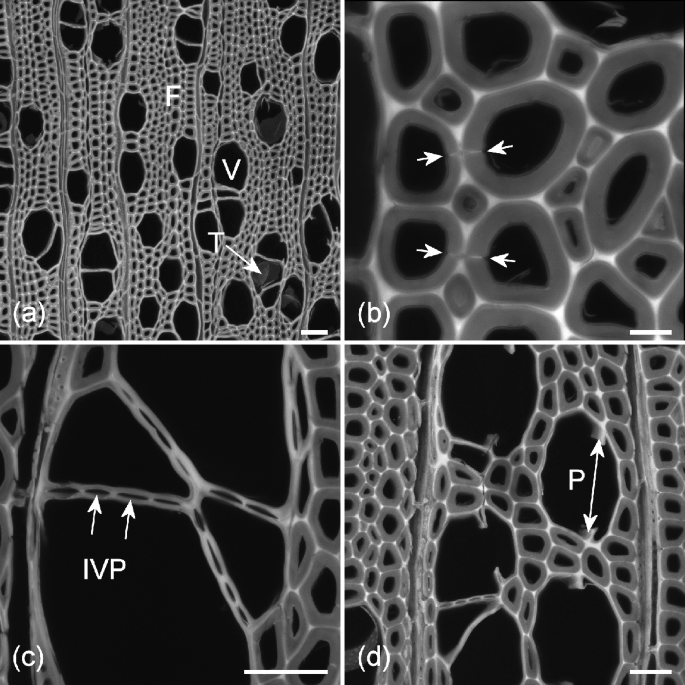The image comprises four black and white sections labeled A, B, C, and D, resembling slides viewed under a microscope. The images feature varying shades of gray and include initials and arrows to identify specific structures, although there are no clear legends or explanations provided. Image A contains initials F, V, and T, while image B has four arrows pointing to unidentified features. Image C showcases the initials I, V, and P with arrows directing the viewer to corresponding parts. Finally, image D includes the initial P, marked in two different areas with interconnected arrows. Each section is separated by thin white lines, and some images contain oval shapes with borders. The exact nature of the images remains indeterminate due to the high magnification and lack of descriptive labels.